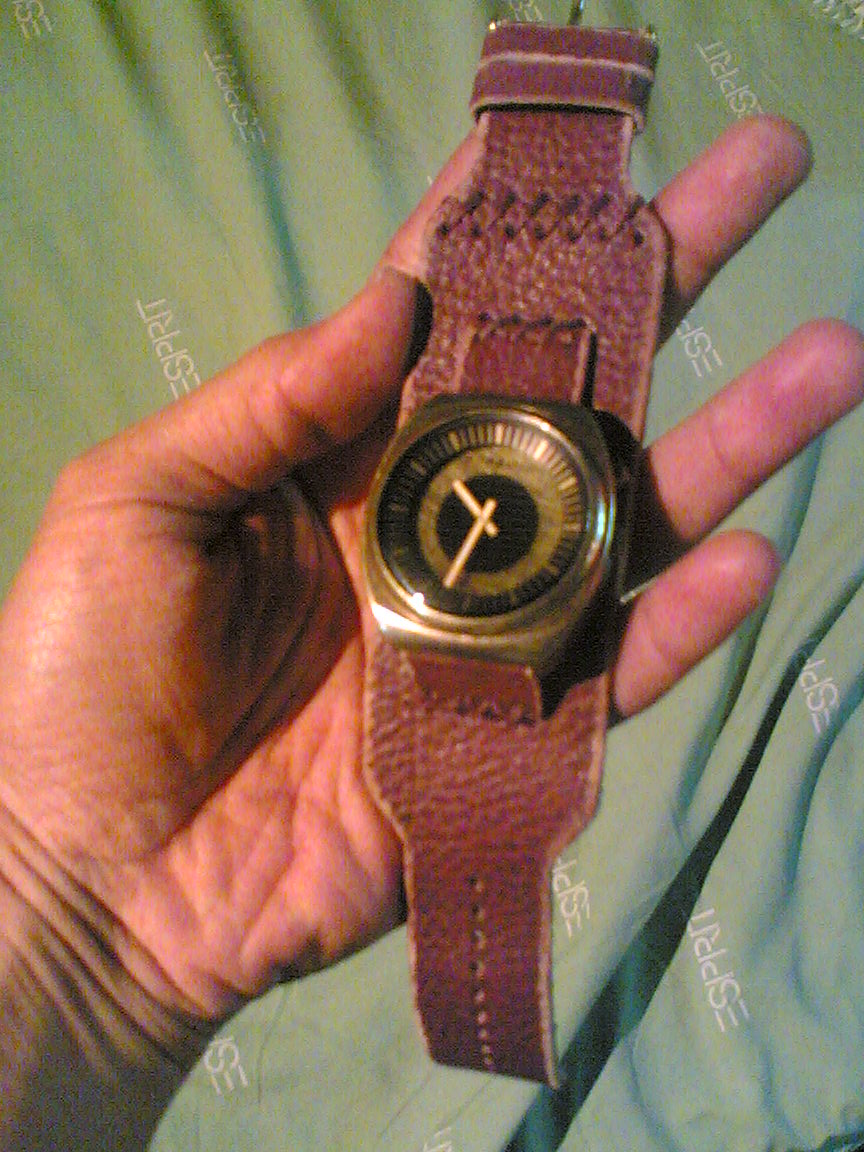This photograph features a man's left hand holding a striking gold watch against a green, wrinkled cloth embroidered repeatedly with the word "Esprit." The fabric is positioned almost upside down, rotated about 100 degrees to the left. The watch, which evokes a 1970s aesthetic, is housed in a cheap, goldish, bronze casing with a round face set within an almost squarish frame. Its face is detailed with minute dashes and thicker bars at five-minute intervals, devoid of numbers. The watch's hands are rectangular and gold, displaying a time of approximately 10:32. The leather strap is notable for its unique design: starting narrow at the watch, it broadens significantly before tapering near the clasp that secures it around the wrist. The strap features thick, brown leather, almost reminiscent of a belt, adding to the vintage charm of the timepiece.